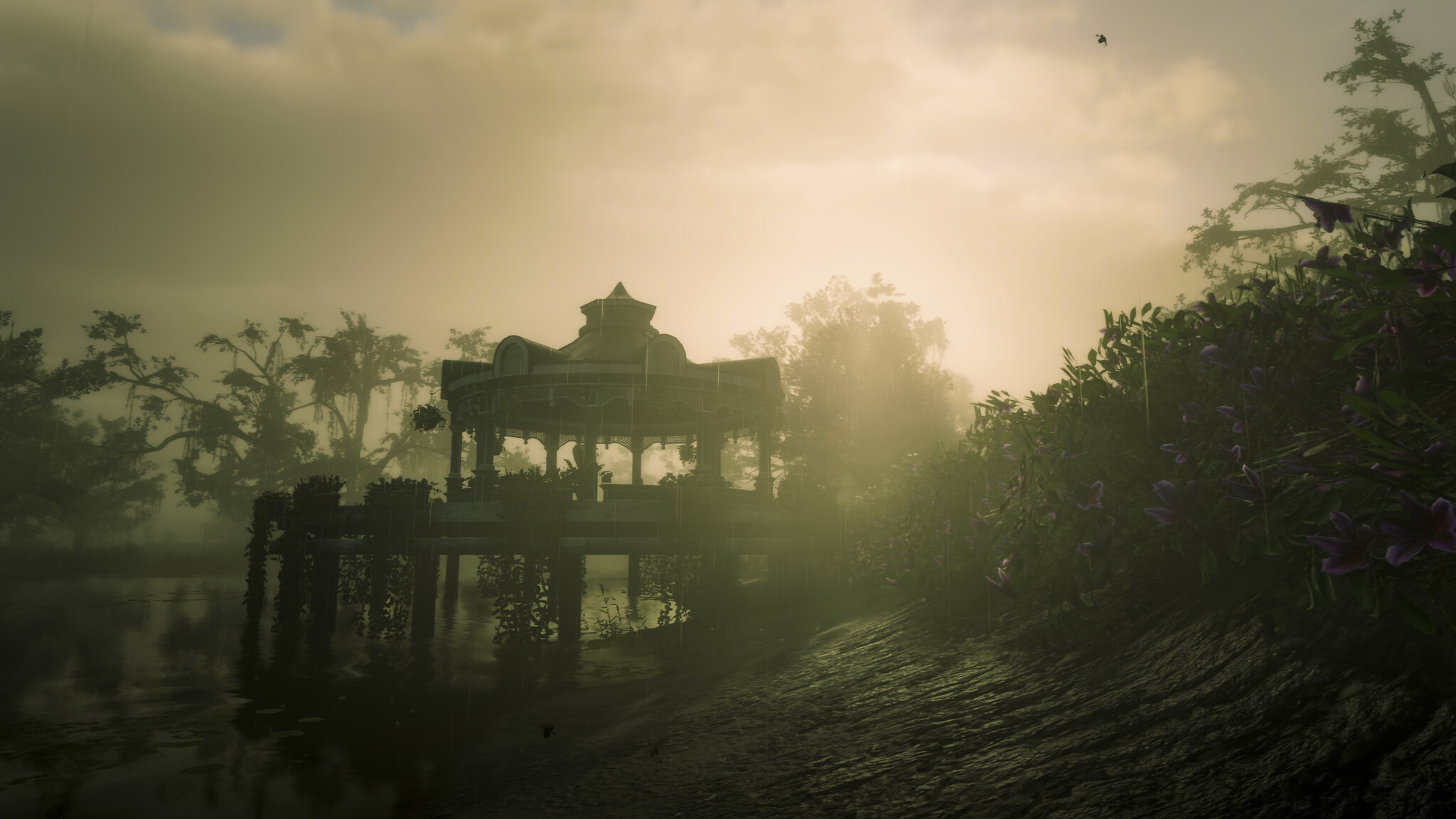Underneath a brooding sky tinged with yellow hues, the heavens are blanketed with a thick layer of dark, gray clouds. Below, waves gently lap against the water’s edge on both sides, framing a serene yet stormy scene. In the foreground, vibrant green leaves dominate a field that extends towards the horizon. Towards the back, an array of trees stands tall, their leaves cascading downwards, creating a lush canopy. The trees' branches fan out, textured with rough bark, adding to the dense woodland feel. To the right, clusters of leaves obscure portions of the view, while visible gaps reveal a background painted in dusky grays. Anchored in the midst of this natural tableau is a wooden platform that supports a charming gazebo, perched tranquilly above a swampy lake or river, inviting contemplation amidst the impending storm.